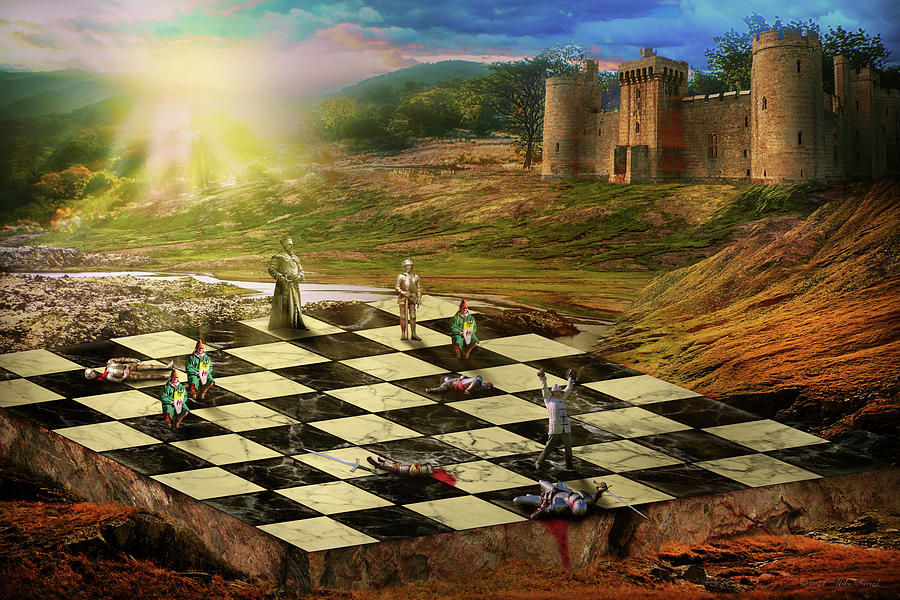The image is a detailed illustration, likely a digital or AI-generated painting, depicting a surreal medieval landscape bathed in vibrant hues of blues, turquoise, pinks, and yellows. A radiant sun on the left casts light over rolling green hills and a lush, grassy area in the foreground. The centerpiece of this landscape is a towering, somewhat worn castle perched on a reddish-clay hill to the right, flanked by various green bushes. At the base of the hill, a river meanders through flatlands, separating the castle grounds from a large black and white checkerboard chess platform dominating the foreground.

The chess platform, designed to accommodate human participants, showcases a dramatic and chaotic scene. Figures in medieval armor, some in victorious standing poses with arms raised, others defeated and lying in pools of blood, are scattered across the board. The scene includes a diverse array of characters: crouching gnome-like figures, a queen-like knight, a contemporary looking figure in a raincoat, jesters in green and red caps, a bishop or king figure, and a celebrating chef character. The juxtaposition of this storybook-like environment with the stark black and white chessboard and lifelike battle elements creates a surreal and visually striking image.